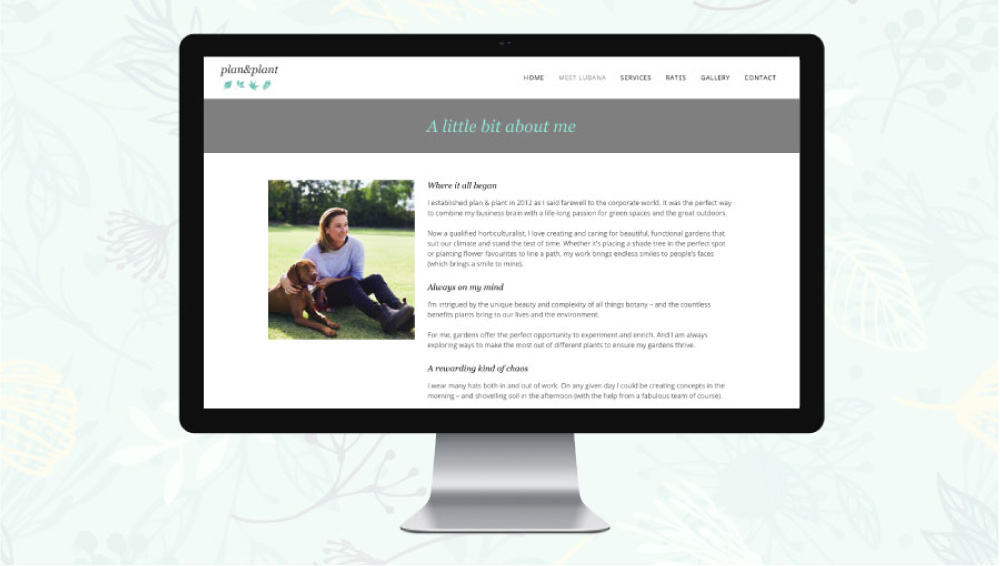Screenshot of a mock-up website displayed on a computer screen. The screen has a black edge with a grey stand at the center bottom, reflecting light. The background features a pale green wallpaper adorned with a pattern of stems and leaves, resembling delicate branches, both behind and below the screen. 

The website's header has a white band displaying the text "Plan and Plant," accompanied by green icons and navigation links, including Home, Visit, Services, Gallery, and Contact. The text on the site is small and somewhat blurry, indicating a non-photorealistic mock-up. 

Central to the website is a section with a grey bar and a heading, "A little bit about me," written in green. Below this heading is an image of a woman with blonde hair, sitting outdoors on grass with a brown dog. She is Caucasian and dressed in a blue top and black jeans. Accompanying the image is text that begins with, "This is where it all began. I established Plan and Plant in 2012." It goes on to describe the founder as a qualified horticulturist passionate about creating and caring for gardens and plants. Despite the difficulty in reading the blurry text, it conveys the founder's dedication to botany and managing various projects.